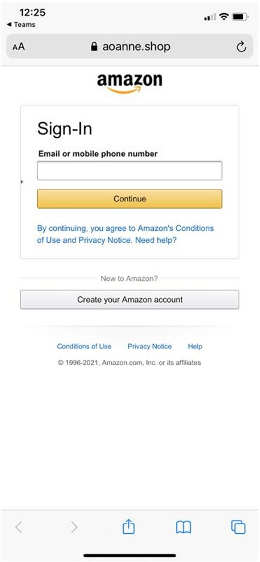The image is a vertically oriented rectangular screenshot, presumably captured from a mobile device. At the very top, there's a light gray status bar. On the left side of this bar, the time is displayed in black text as "12:25." Moving right, the status bar shows various icons including a cell phone signal indicator with two out of four bars, a fully filled Wi-Fi signal, and a battery symbol that appears to be approximately 75% charged.

Beneath the status bar, a black left-pointing arrow is visible, accompanied by the text "Teams." Below this, there is a darker gray navigation bar. Within this bar, a lock icon is centrally located beside the text "aoanne.shop" and a refresh symbol on the far right.

A thin dividing line separates this navigation bar from the main content of the screenshot, which features the Amazon login page. The Amazon logo, with its emblem, sits at the top. Below the logo, there is a text field labeled "Email or mobile phone number" outlined in gray, but the field itself is currently blank. An orange button with black outlined text that says "Continue" is immediately below the blank text field.

Further down, a disclaimer in blue text reads, "By continuing, you agree to Amazon's Conditions of Use and Privacy Notice." and "Need help?" Below this, written in very light gray font, is the phrase "New to Amazon?" flanked on either side by thin lines.